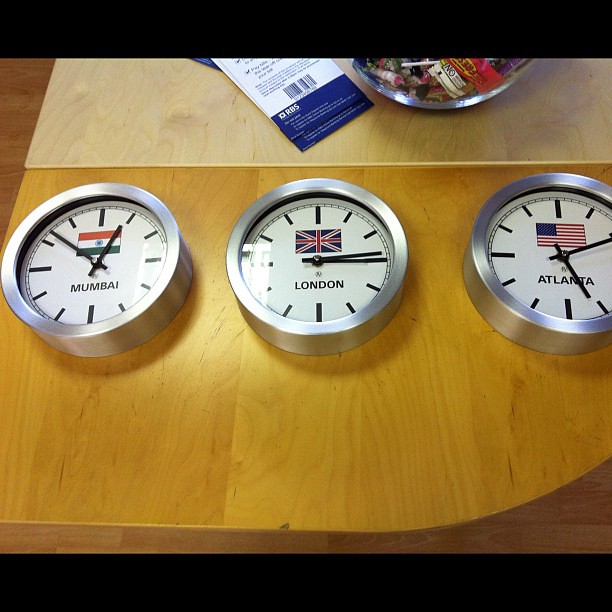This photograph captures a distinctive wooden table, notable for its two-tone design. The table features a light blonde stain on one side and a contrasting honey stain on the other, both outlined by a darker brown border along the edges. Positioned on this table are three identical clocks, each encased in a silver frame with a white clock face. The clocks, designated for Mumbai, London, and Atlanta, each display the corresponding country flag beneath the 12 o'clock position. The clocks are designed with black hands and minimalistic black lines in place of numbers, with smaller notches indicating the minutes.